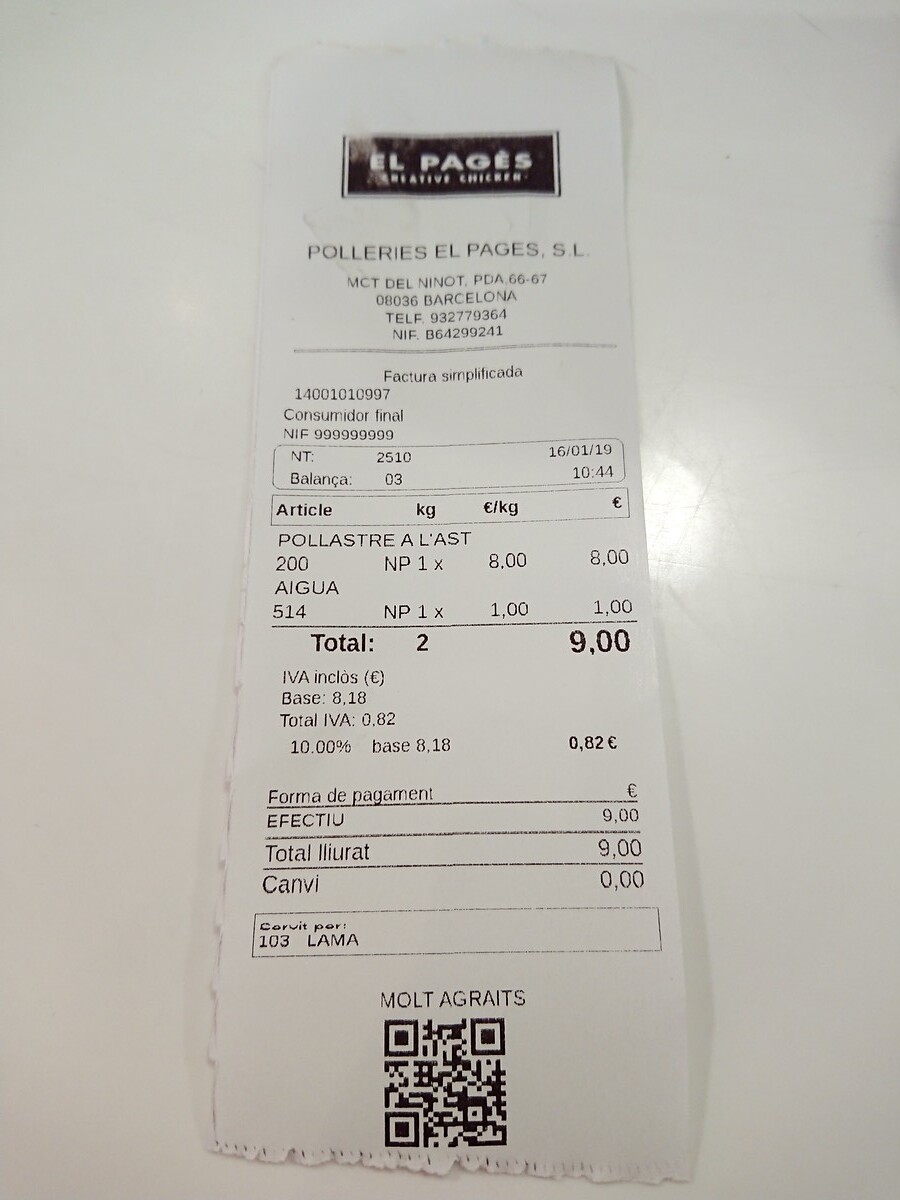The image showcases a white restaurant receipt with black text from El Pajes Creative Chicken, located in Barcelona, as indicated by the address and phone number. The receipt features the name "Pollieres El Pajes S.L." near the top, just below the restaurant name. The transaction date is 16-01-19, and it was completed at 10:44 AM. The receipt lists two items: "Pollastre" (likely chicken) costing 8 euros and water for 1 euro, making the total 9 euros. The receipt details the tax calculation but confirms the total remains 9 euros. Notably, the order number is 103, and a QR code is present at the bottom. The receipt is photographed on a reflective white surface, possibly a table or cutting board, adding to the image's monochromatic appearance.